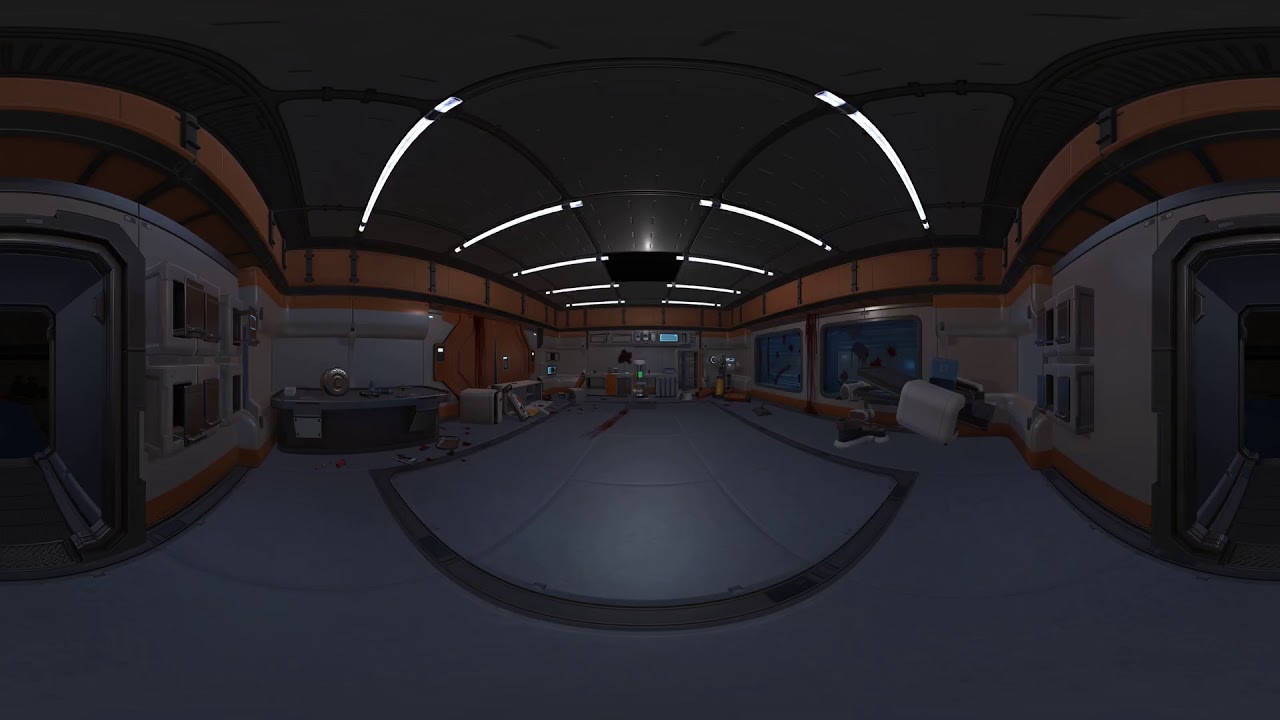The image appears to be a detailed, high-resolution screenshot from a futuristic video game, possibly "Dead Space," depicting a scientific research facility or space station. The room is adorned with advanced, futuristic equipment and features a blue floor, gray walls with orange trim, and a black ceiling illuminated by long fluorescent tube lights. The setting exudes a sense of unease, possibly due to a violent incident, evidenced by the disarray and debris scattered across the floor. On the right, part of a doorway is visible leading to another room with windows that offer a glimpse inside, though details are obscured. Additionally, a workbench cluttered with robotics and isolation pods for experiments can be seen, along with a two-way glass mirror, creating an environment ripe for exploration within this virtual reality or video game space.